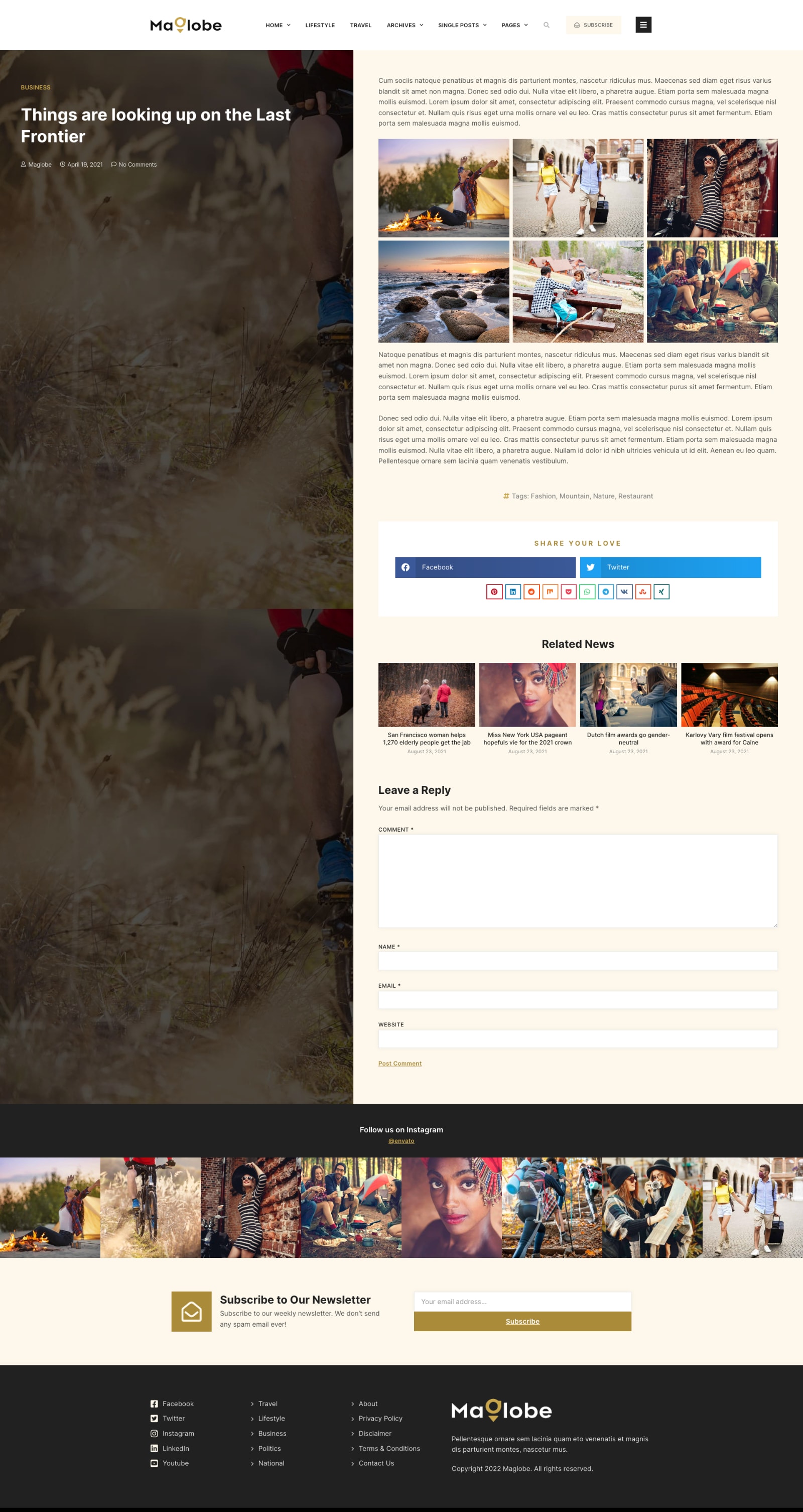The image showcases a web page from "My Globe." At the top left corner, the words "My Globe" are written, with "My" and "Globe" split by a brown globe icon. The page is zoomed out, rendering the text quite small. On the left side of the page, there is a white-text heading stating "Things are looking up on the last frontier." The background features an image of dry, brown grass.

On the right side, there’s an article that isn't easily readable owing to the small text size. The article includes various pictures: people camping, holding hands, swimming, enjoying a lakeside, sitting in a circle, and working across desks from each other. Below the article, social media sharing icons for Facebook (blue) and Twitter (light blue) are present, with the prompt "Share your love."

Towards the bottom of the page, under "Related News," there are additional articles with accompanying small images. A comment section titled "Leave a reply" follows, with space provided for users to submit their comments. The page also invites users to "Subscribe to our newsletter," offering a field for email input and a brown "Subscribe" button. The footer of the page reiterates "My Globe" with some additional, unreadable text.